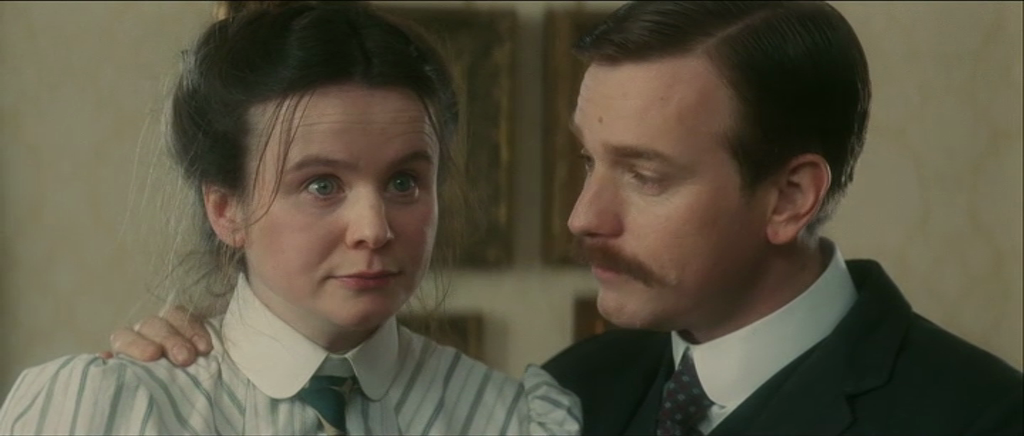The image appears to be a cinematic or staged scene set indoors, possibly from a movie or a show, with an old-fashioned ambiance. It features a close-up of two people standing in front of a beige or white wall adorned with four thick, gold-bordered picture frames. The man, positioned on the right side, wears a gray suit jacket over a white, rounded-tip collared shirt and a brown tie with blue polka dots. His slicked-back, perfectly parted black hair and prominent long mustache give him a distinguished appearance. He places his right hand on the woman’s shoulder, who stands on the left. The woman exudes a sense of frazzled fear, her blue eyes wide open as she gazes slightly towards the unseen figure she's facing. She wears her hair in a slightly disheveled bun, with strands falling loosely. Dressed in a white button-down shirt with gray pinstripes, she also sports a green collared tie, and a green jacket, adding to her distressed yet formal look.